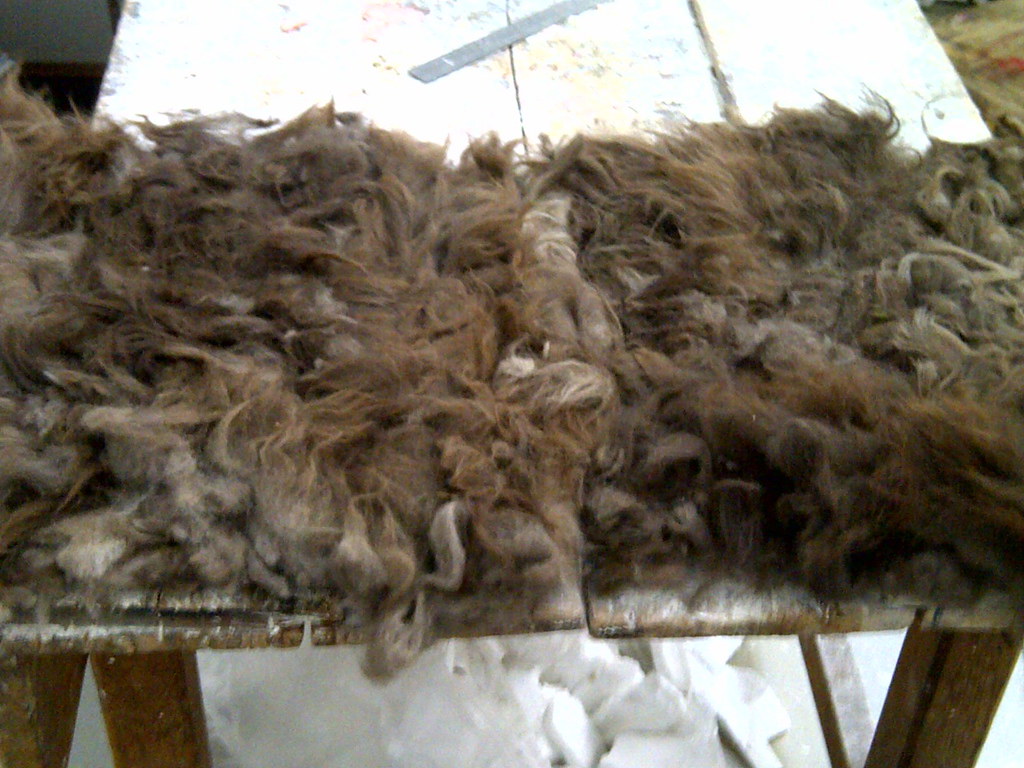The photograph captures an outdoor setting with a weathered wooden table covered in a large pile of unprocessed wool from sheared sheep or goats. The wool varies in shades, from dark brown to light tan, grayish brown, and light gray. Beneath the table, wide white wooden slats, reminiscent of a picnic table, are visible, suggesting the scene is outdoors. In the upper right-hand corner, there's a blurred patch of something green, likely grass or a flower, while the top left is cast in shadow, adding a dark, gray tone. The wool appears uncleaned, with its original, uncarded state spread out across the table, indicating the aftermath of shearing. The poorly taken, low-resolution image hints at the rustic nature of the setting.